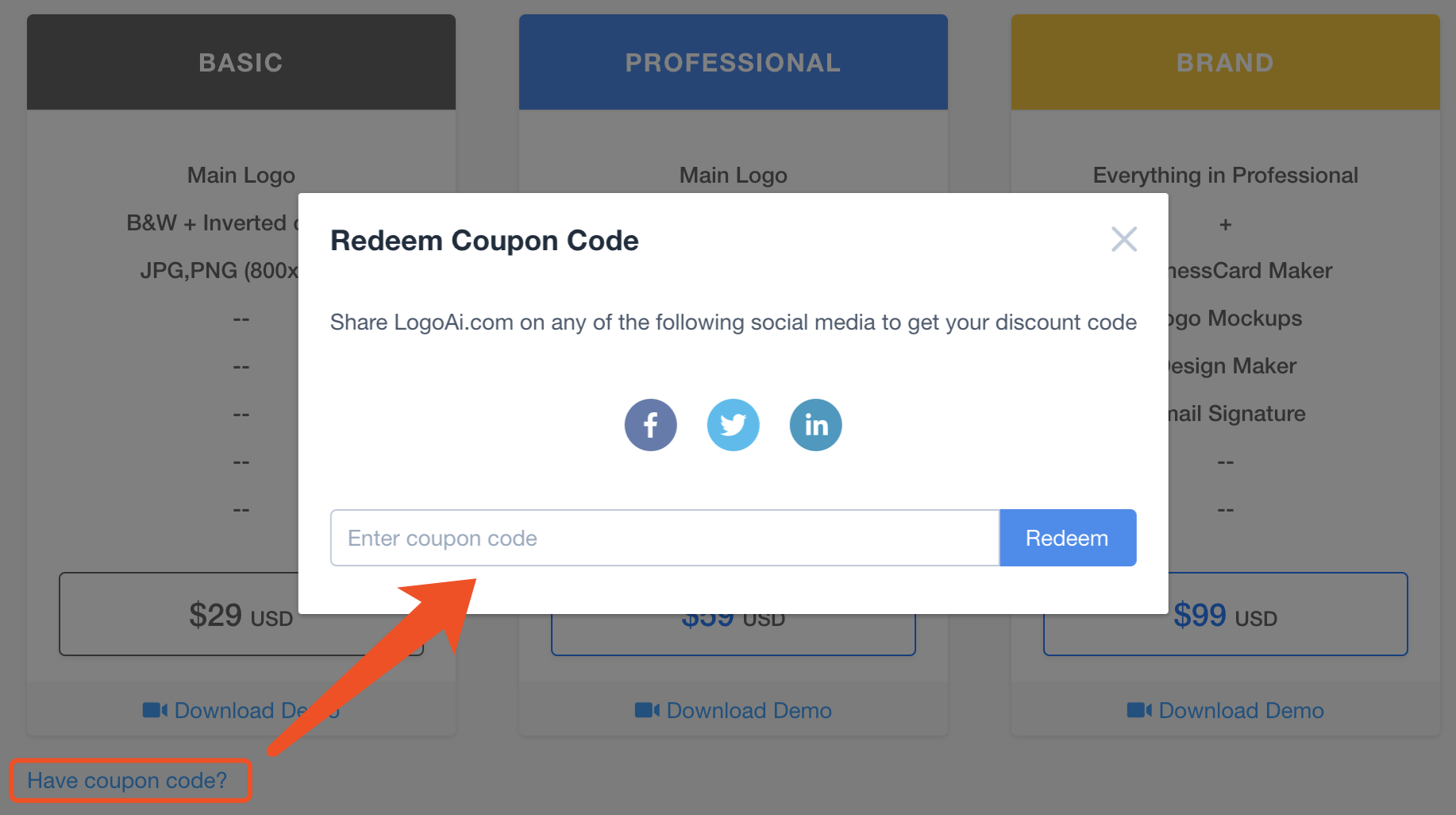In this screenshot, we are viewing the interface of a website that offers three programs, organized from left to right. Each program is highlighted with distinct pricing and features. 

1. **Basic Program**:
   - The primary logo of the Basic Program is displayed in a black and white inverted style.
   - The price is marked at $29 USD, highlighted in orange.
   - Below this, there is an orange arrow pointing towards a white box labeled "Redeem coupon code" in black bold text.
   - In the upper left corner of this section, it instructs users to "Share logoAI.com on any of the following social media to get your discount code."
   - Beneath this, three round icons are shown, representing Facebook, Twitter, and Instagram.
   - There is an open box for entering a coupon code with a blue button labeled "Redeem" alongside it.

2. **Main Program**:
   - Labeled with the Main Program’s logo.
   - To its right, a yellow banner reads "Brand."
   - The cost is listed as $99 USD.
   - Beneath this is a clickable option to "Download demo."

Overall, the webpage uses a combination of bright colors such as orange, blue, and yellow to highlight interactive elements, making it intuitive for users to find and redeem discount codes, and to access program demos.